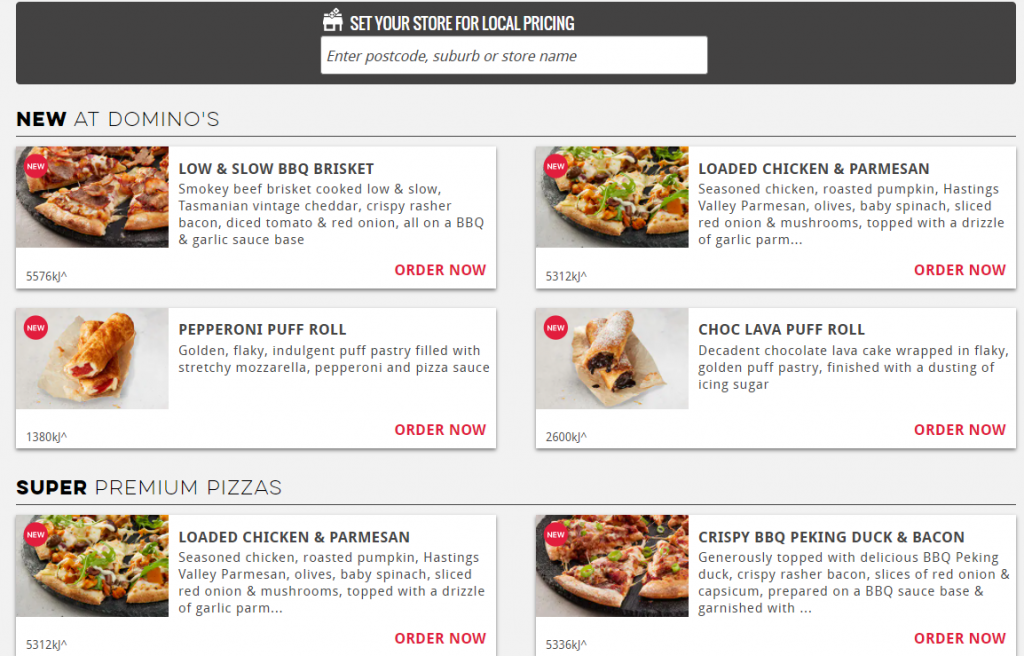The image appears to be a detailed capture of a promotional webpage for Domino's, showcasing various new menu items. 

At the very top, there's a gray banner featuring a white font that reads, “Set your store for local pricing,” accompanied by a small business icon. Below this banner is a search bar prompting users to "Enter postcode, suburb or store name."

The main section highlights several mouth-watering new items:

1. **Low and Slow BBQ Brisket Pizza**: This item is depicted with a tantalizing image of a pizza. The topping consists of smoky beef brisket cooked low and slow, Tasmanian vintage cheddar, crispy rasher bacon, diced tomato, and red onion, all layered on a BBQ and garlic sauce base. A prominent red “Order Now” button is present.

2. **Pepperoni Puff Roll**: Shown with an image of golden, flaky puff pastry filled with stretchy mozzarella, pepperoni, and rich pizza sauce. The appearance hints at a gooey, indulgent filling with an inviting texture. The description highlights the golden crust and appetizing cheese.

3. **Super Premium Pizzas - Loaded Chicken and Parmesan**: This pizza includes seasoned chicken, roasted pumpkin, Hastings Valley Parmesan, olives, baby spinach, sliced red onion, and mushrooms, all topped with a drizzle of garlic Parmesan sauce. The image features a gold crust with visible garnishes that enhance its visual appeal.

4. **Choc Lava Puff Roll**: This decadent dessert is portrayed with flaky golden puff pastry encasing a rich chocolate lava filling, finishing with a dusting of powdered sugar. The image shows dark, molten chocolate oozing out, appealing to any sweet tooth.

5. **Crispy BBQ Peking Duck and Bacon**: This final item, although its full description is cut off, includes generous toppings of BBQ Peking duck, crispy rasher bacon, slices of red onion, and capsaicin on a BBQ sauce base. The image reveals a beautifully garnished pizza with a flaky crust.

In each detailed bullet point, Domino’s encourages immediate indulgence with a clear red “Order Now” call to action, ensuring that the presentation is as mouth-watering as possible.